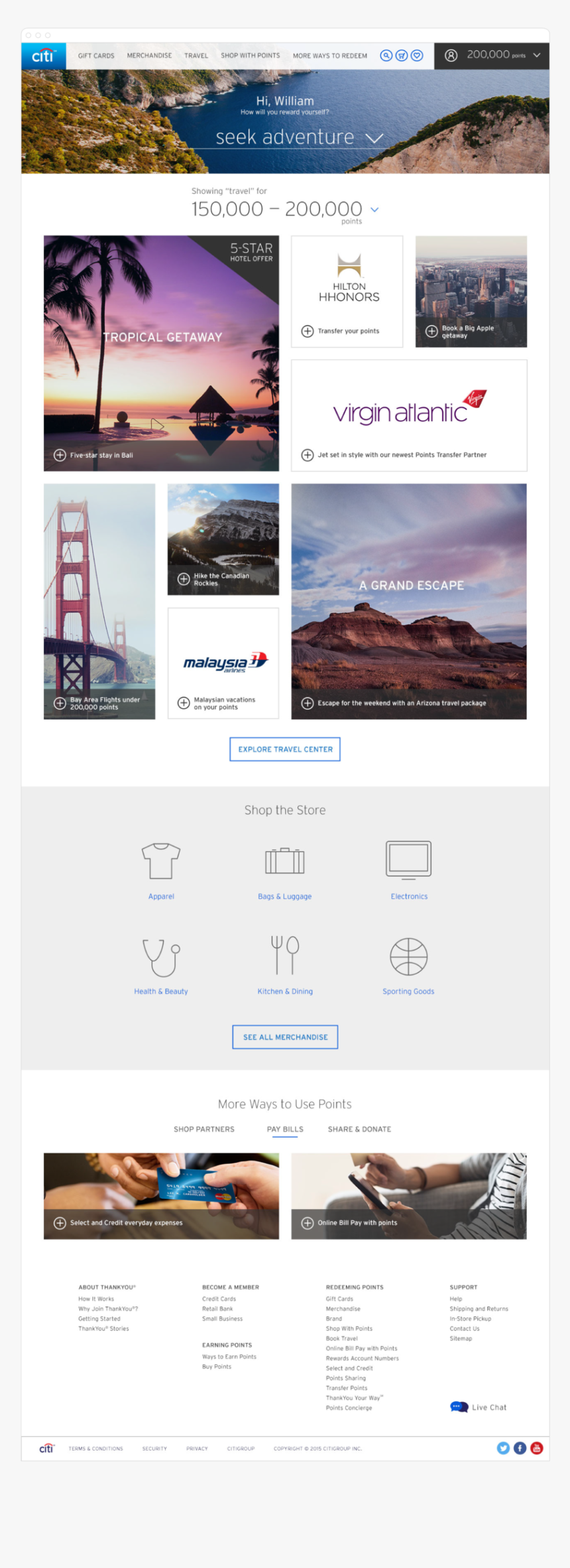A screenshot of a vibrant, adventure-themed website featuring an island setting surrounded by water. The main focus highlights the enticing call to "Seek Adventure" with intricately decorated typography, although the text is relatively small. It also showcases several images including another island with more urban features, a cityscape, a stunning bridge, a picturesque town, and multiple majestic plateaus. Overlaying the plateaus is the inspiring text "Grand Escape." Additionally, the bottom section of the screenshot displays a picture of a couple holding what appears to be a credit card, and another image of a man lounging on his couch while using his phone. The text mentions figures ranging from 150,000 to 200,000, possibly indicating a user count or adventure options. Various logos including "Virgin" and "Atlantic" are also visible, suggesting partners or themes related to travel and exploration.